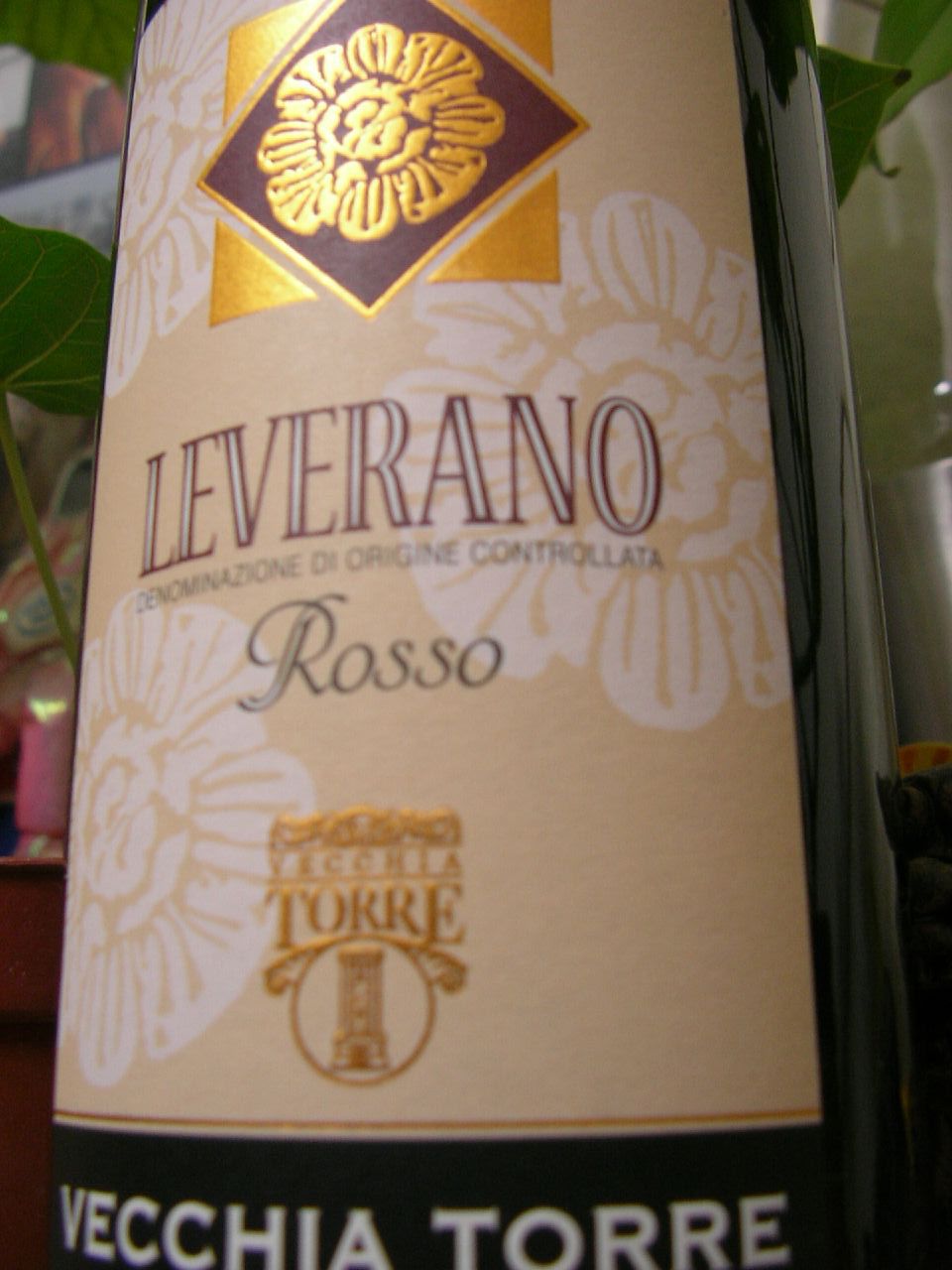This is a close-up of the label on a bottle of wine or some type of liquor, surrounded by a soft, plant-filled background that adds a natural, flowerish ambiance. The label itself is primarily beige adorned with white flowers, giving it an elegant and refined appearance. At the top of the label, there's a notable maroon diamond with a golden flower emblem within it, enhancing its visual interest. This diamond is further set against a gold square, emphasizing its significance. 

The central text on the label reads "Leverano" in a combination of maroon and white, followed by some smaller text in a language that is not identified. Below this, the word "Rosso" is displayed prominently in black. Additionally, there are two notable gold emblems on the label - one in the middle and one towards the bottom. The name "Vecchia Tori" appears twice in gold script, once just below the central text and again at the bottom in white on a black background, likely indicating the producer's name. This detailed and decorative label suggests a classic and possibly premium quality, resonating with the elegance of traditional wine labeling.